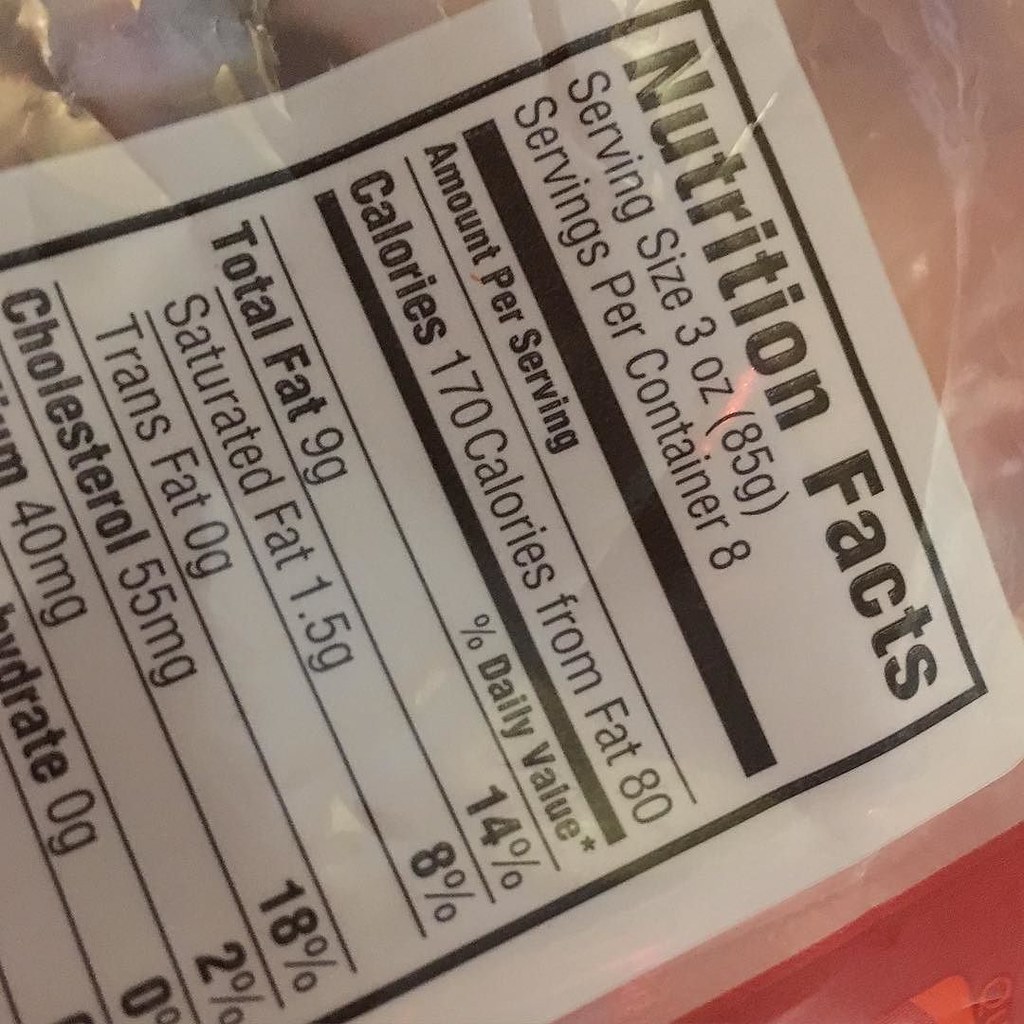This is a close-up photograph of a Nutrition Facts label on a food product packed in a transparent plastic bag. The label is a white sticker featuring black lettering and a black border, and it is placed at an angle around 70 degrees from vertical. The label details include: "Nutrition Facts" in bold, a serving size of 3 ounces (85 grams), with 8 servings per container. Each serving contains 170 calories, with 80 calories from fat. The total fat content is 9 grams, representing 14% of the daily value, of which 1.5 grams are saturated fat (8% daily value) and 0 grams are trans fat. Additionally, it lists 55 milligrams of cholesterol, 40 milligrams of sodium, and 0 grams of carbohydrates. The layout of the label is structured, with each category separated by black lines, creating an appearance similar to lined paper. There is a hint of red and pink hues along the right side of the image, likely due to lighting or reflections from the packaging.